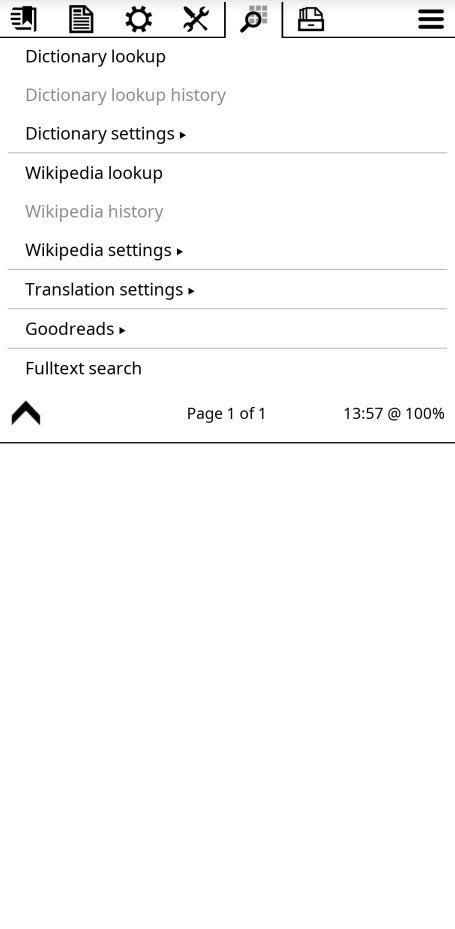In the upper left corner, the image features a series of horizontal lines next to a longer vertical black box. To the right of this, there is a small section that resembles a piece of paper, about an inch high, with black horizontal lines across it. Continuing further to the right, there is an icon that looks like a settings wheel, followed by overlapping images of a wrench and a screwdriver. Just beside these tools, there is a small magnifying glass icon.

Below this series of icons, on the left side, the text reads "Dictionary Look Up," followed by "Dictionary Look Up History," and "Dictionary Settings," with an arrow pointing to the right. Below this text, there is a long horizontal line. Further down, the text reads "Wikipedia Look Up," "Wikipedia History," and "Wikipedia Settings," followed by another long horizontal line. Further still, it reads "Translation Settings," followed by yet another line, "Goodreads" and "Full Text Search." 

On the bottom-left corner, there is a black arrow pointing upward. To the right of this arrow, it says "Page 1 of 1." Finally, in the bottom-right corner, it reads "13:57" and "100%."